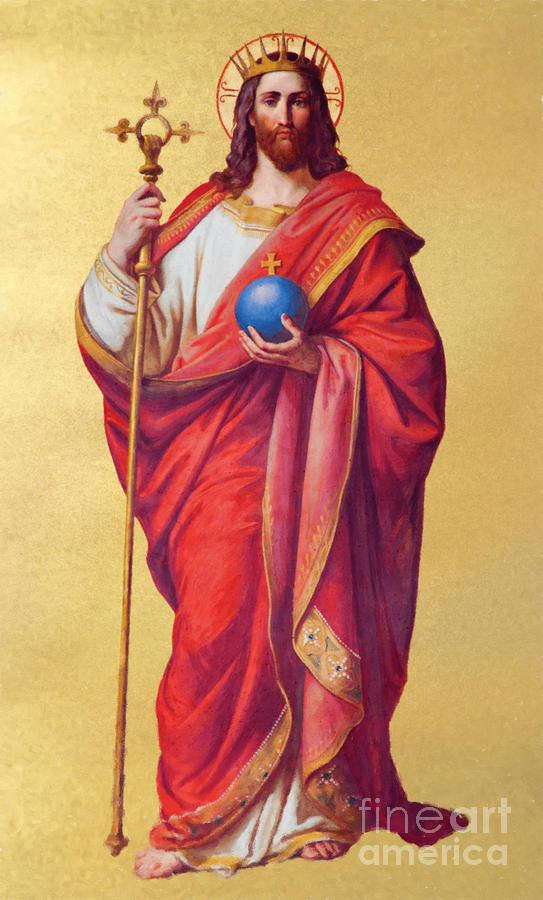This is a detailed, elegantly drawn depiction of Jesus Christ, set against a yellow backdrop. Jesus is portrayed with long brown hair, a reddish-brown beard, and a gold crown on his head. A red halo-like circle is behind his head, adding a sacred aura. He is dressed in a flowing red robe with yellow frills, draped over a white gown with gold accents around the sleeves and neck. In his left hand, Jesus holds a large blue orb featuring a gold cross. His right hand grasps a gold staff adorned with three fleur-de-lis and a circular design. He is barefoot, standing solemnly and gracefully. The bottom right corner of the image bears a white, bold inscription: "Fine Art America."